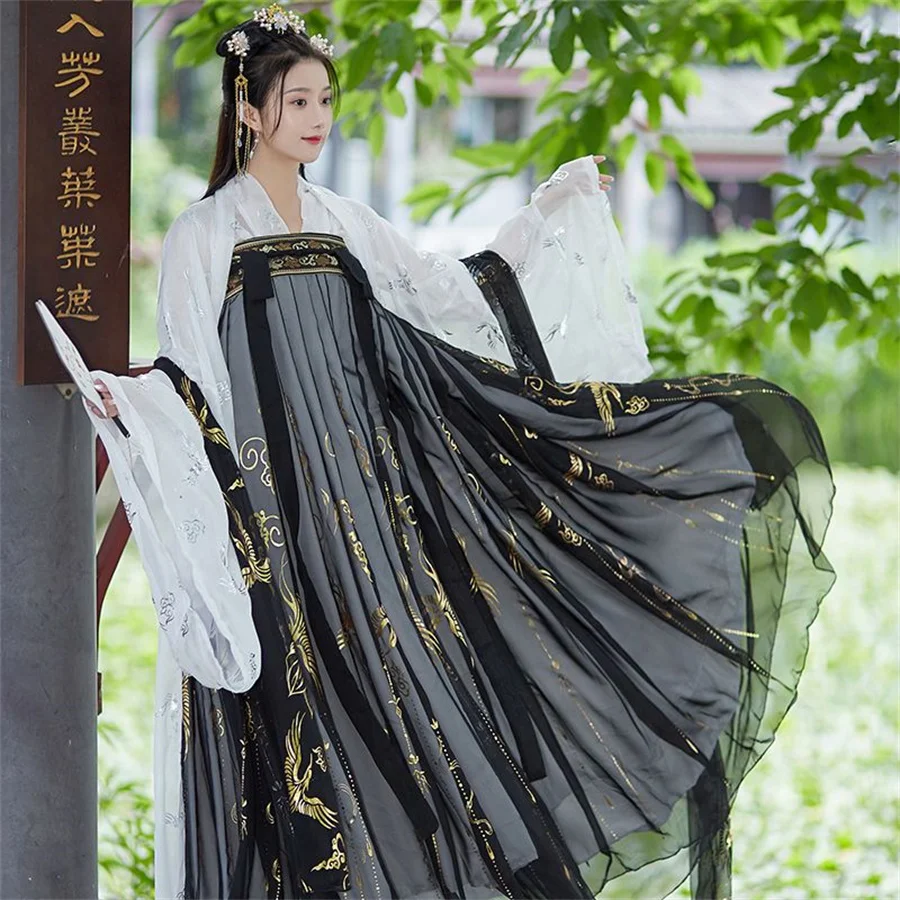A captivating photograph showcases a young Asian woman with ivory skin and black hair adorned with white and gold flower decorations. Her hair is elegantly tied up, complemented by little bows and ribbons. She is dressed in a flowing, traditional Chinese outfit featuring a big, billowy white top with loose sleeves and a long black skirt. The top is connected at the chest by a black band intricately embroidered with gold and brown designs, including delicate birds. She holds a hand fan and stands next to a gray wooden post with gold-engraved Chinese lettering. The background reveals lush green trees and grass, suggesting a serene outdoor setting on a beautiful day. The woman exudes a calm and elegant aura, looking off to the right with a blank expression.